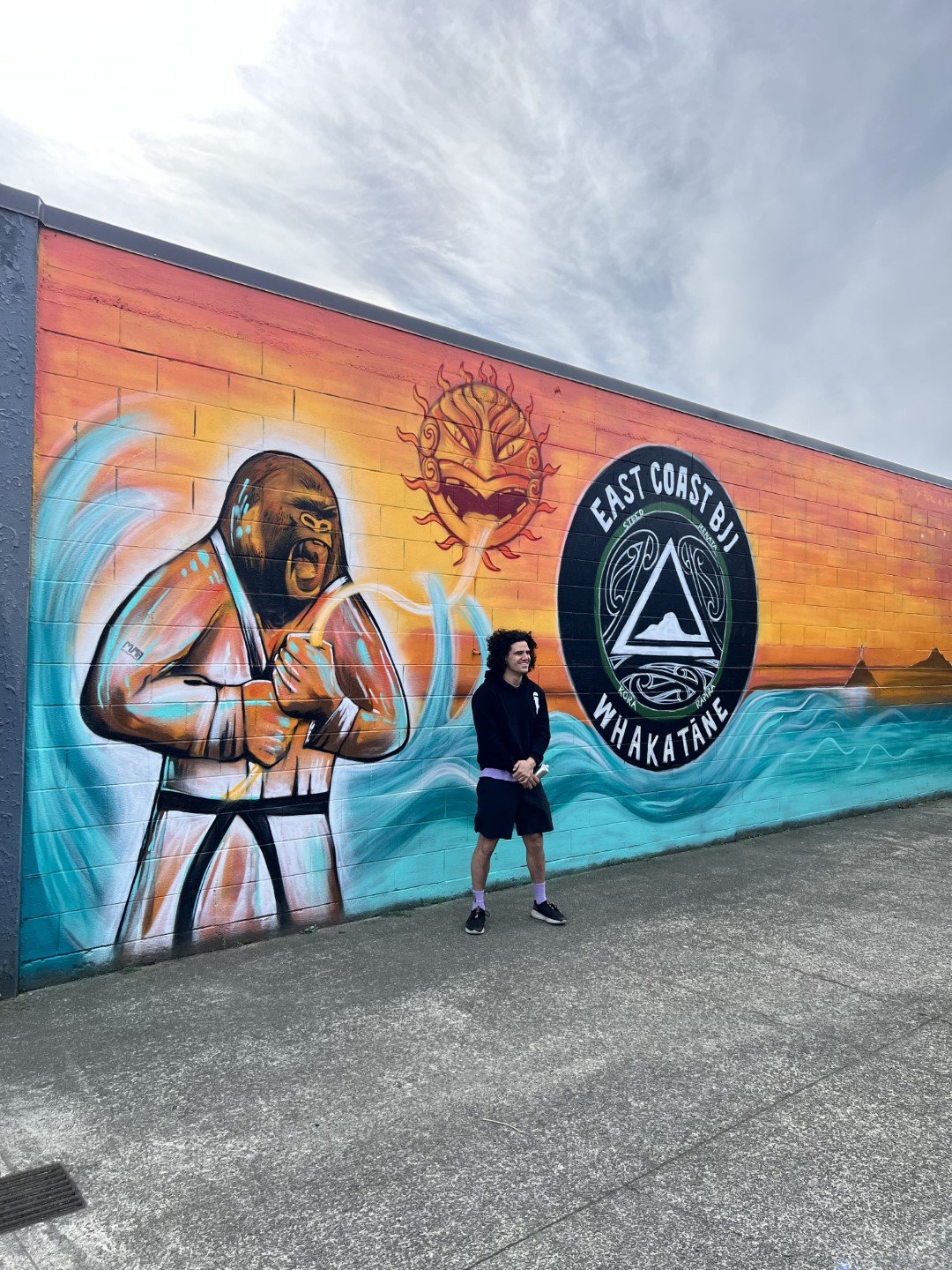A young man stands against a vivid, expansive mural painted on a brick wall. He is dressed casually in a black hoodie over a gray t-shirt, black shorts, white socks, and black sneakers. In his hand, he holds a water bottle. The mural behind him is vibrant and detailed, showcasing a dramatic scene. Central to the artwork is a gorilla clad in a white karate outfit with a black belt, gripping the extended tongue of a monstrous sun, which has a furious, demonic expression. Surrounding the gorilla is an ocean scene with splashing blue water. The sky depicted above transitions from a bright yellow-orange sunset to a blue-gray with wispy white clouds. Prominent on the mural is a large black circle featuring the words "East Coast BJJ" and "Wakatane" with a white triangle emblem in the center. The mural's ground level shows a concrete surface extending outward.